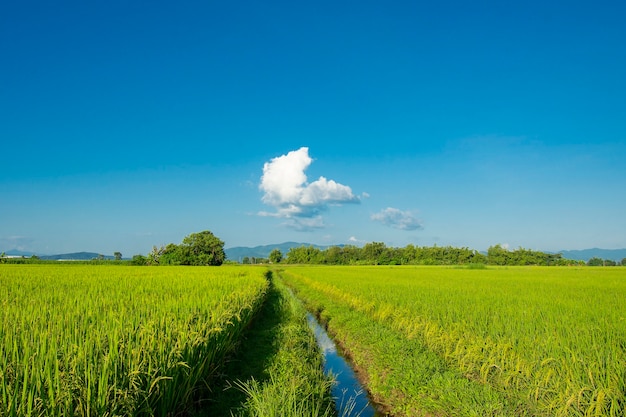In this photograph, we are presented with a lush agricultural field, likely filled with a tall and slender grain crop, which could be rice or wheat. The field is bisected by a narrow drainage ditch, reflecting a vivid blue sky scattered with a few puffy white clouds. This scene exudes vibrant shades of green from the crops and varied tones of blue from the sky, fading to almost white near the horizon.

The ditch, resembling a small stream, has been accentuated by the pristine reflection of the clouds and sky in its water. Alongside the field runs a walking path with neatly mowed grass, around six feet wide. In the background, a row of trees stands tall, and beyond them, faint mountain peaks can be discerned.

The upper half of the photograph is dominated by the vast, clear blue sky, melting into the light blue of distant mountain ranges. This picturesque scene, rich with natural beauty, captures the essence of a serene, sunny day with a harmonious blend of greens, blues, and whites.